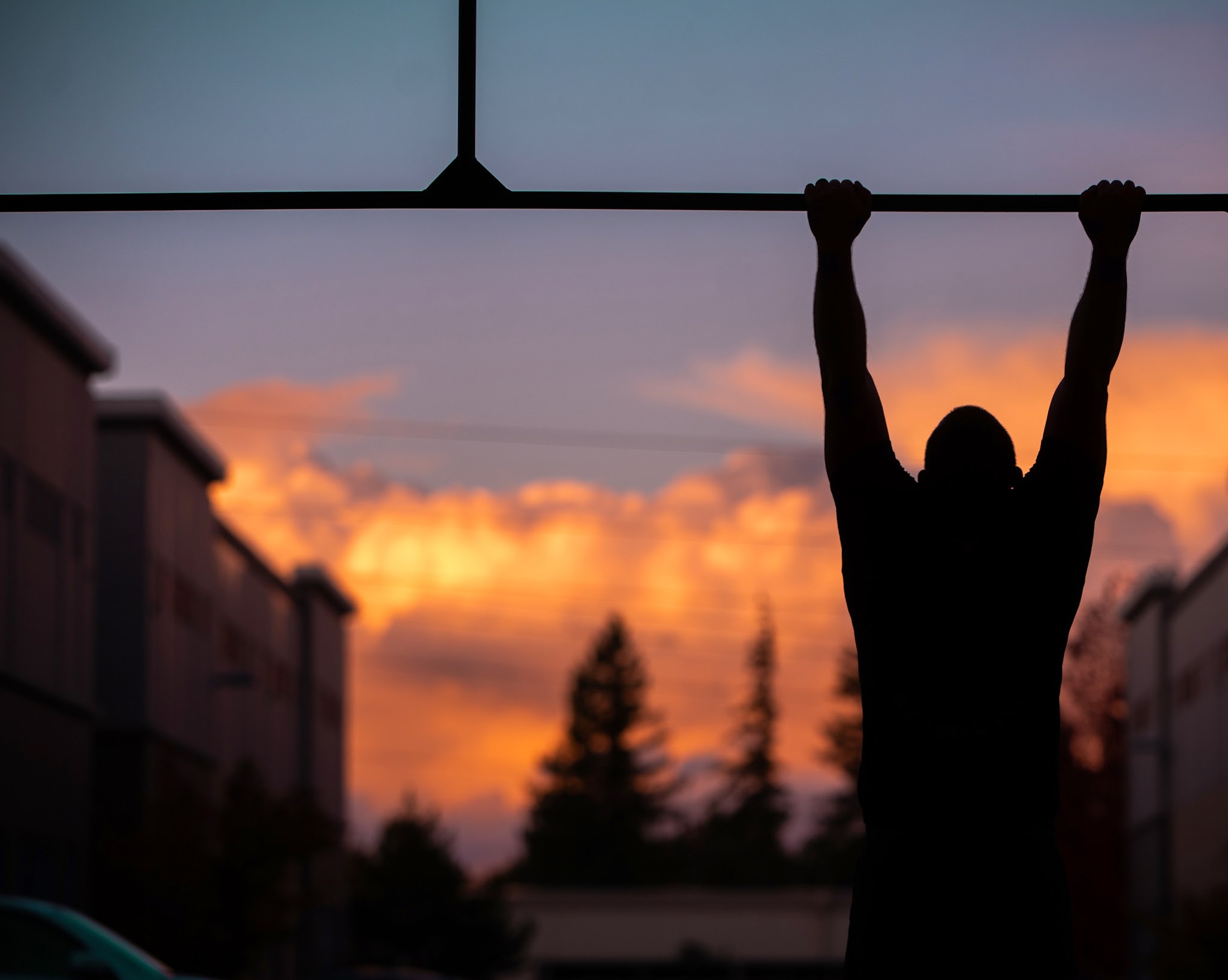In this captivating sunset scene, a muscular, bald man is seen gripping a makeshift bar, possibly performing pull-ups or hanging in a workout session reminiscent of a "rocky-esque" use of urban surroundings. His body is silhouetted against a vibrant backdrop of glowing orange, gold, yellow, and purple hues, with the sky transitioning to dark gray above the colorful clouds. The man's arms hang straight as he faces forward, his distinct physique evident. On either side of him, silhouettes of apartment buildings or townhomes frame the image, while large pine trees and indistinct foliage are visible in the background. The entire scene conveys a sense of peaceful determination at dusk, blending the raw beauty of the sunset with the man's rugged workout routine.